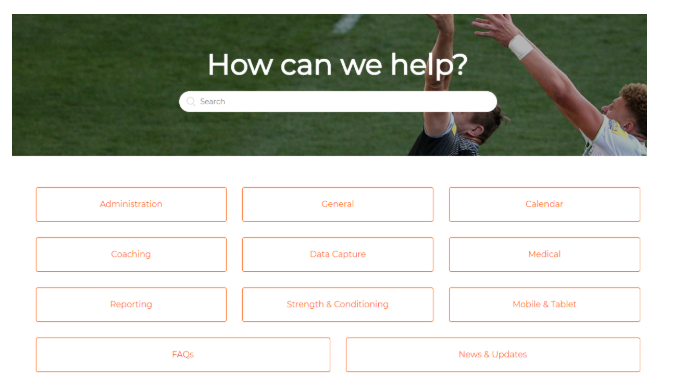In this image, set against a stark white background, a screenshot of a web page is depicted with meticulous detail. The top third of the page features a large banner photo showcasing lush green grass and two individuals reaching their left hands upward. Positioned to the right within this banner, the first person, situated in the lower-right corner, is partially visible from the shoulders up. This individual, assumed to be a man, has fair skin, curly hair, and is clad in a white t-shirt, captured in profile. Directly in front of him, another man with dark hair, also raising his left arm, is wearing a dark t-shirt. To the left of their upward-stretched arms, in bold white text, the phrase "How can we help?" is prominently displayed. Below this text sits a clean, simple white search bar designed for user inquiries.

Following the banner section, nestled against a white background, is an array of functional buttons structured into rows. The top row, aligned to the left, comprises three buttons labeled "Administration," "General," and "Calendar," each characterized by a white hue and outlined in a soft peach color. Directly below, in the subsequent row, three more buttons labeled "Coaching," "Data Capture," and "Medical" are similarly designed, maintaining a cohesive and user-friendly interface.